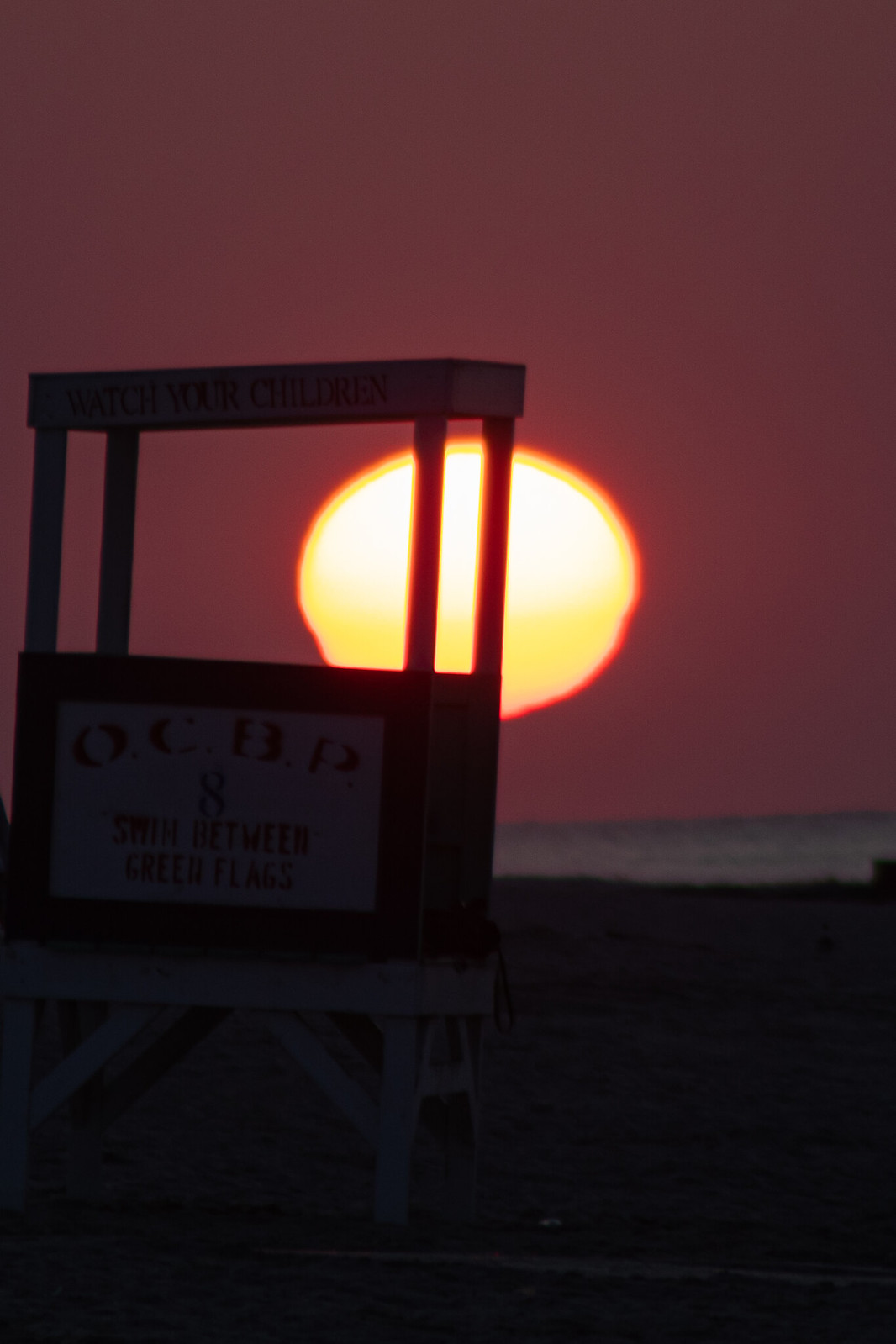The image captures a serene beach scene at sunset. The sky is predominantly dark gray to black at the top, transitioning to a pink and reddish hue with the sun, which has a red outline with an orange bottom and white top, positioned in the center above the water. The calm water itself reflects the red hues of the sky, adding to the tranquil ambiance. Below, the beach is covered with a white substance that could be either snow or sand. On the left side of the image stands a small wooden lifeguard station or cabin, marked with "OCBP-8" and a notice that reads "Swim between green flags." This structure has a simple roof and is supported by four wooden poles, resembling scaffolding. The detailed wooden surface and the rugged terrain add texture to the foreground, enhancing the rustic and peaceful vibe of this coastal sunset.